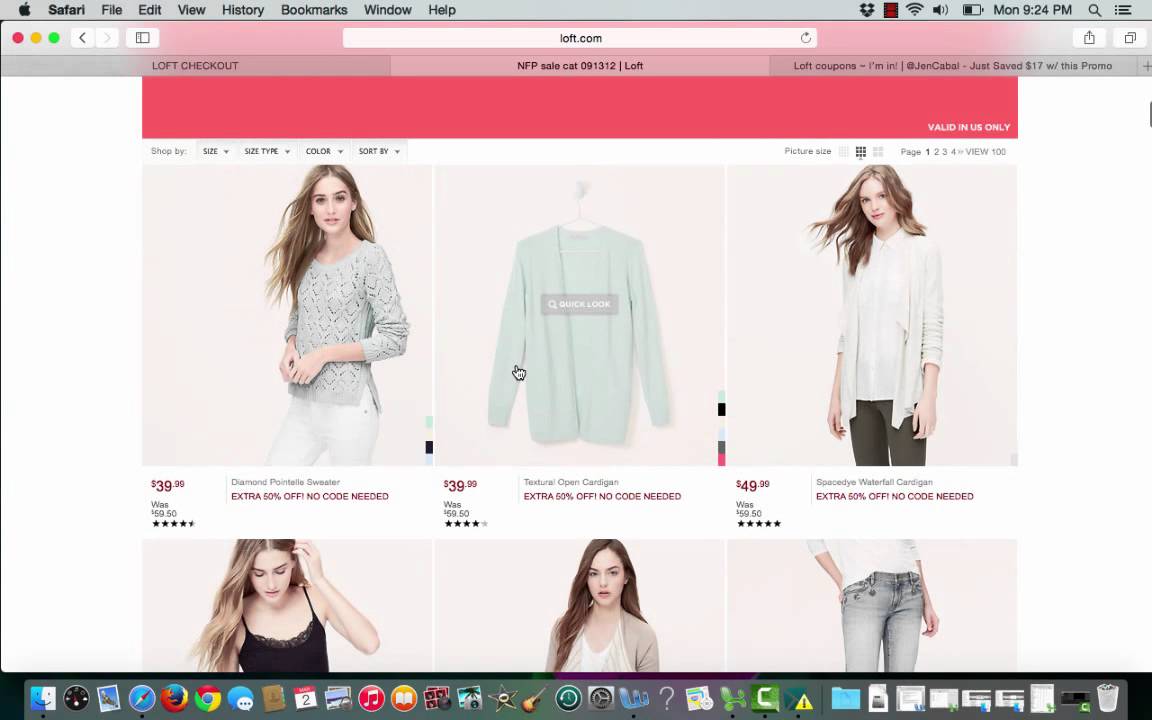Screenshot of LOFT Clothing Store on Apple Mac Computer

This image captures a screenshot taken on an Apple Mac computer, specifically showcasing the interface of the clothing store website, Loft.com. The familiar Apple menu bar is visible at the top with options including Safari, File, Edit, View, History, Bookmarks, Window, and Help presented in grey and black fonts. The taskbar at the bottom of the screen displays a variety of icons representing different applications typically found on a Mac.

The website being viewed, loft.com, is prominently displayed and has a clean, predominantly white design with pink accents. The red, amber, and green dots characteristic of Mac windows are visible at the top left corner of the browser, indicating the window's control buttons.

Central to the screenshot are six images that showcase different female clothing items. Four of these feature models wearing various outfits:
1. A model dressed in a top and shorts.
2. Another model sporting a top and pants.
3. A partially visible model in bedwear, wearing a cardigan and top.
4. A highlight on jeans worn by a model.

Additionally, one image presents a single jumper on a clothing hook, emphasizing the item on its own.

The website's visual layout is designed to be easy on the eyes, utilizing a soft color palette of pink and white tones against the clean background, drawing focus to the fashion pieces displayed.